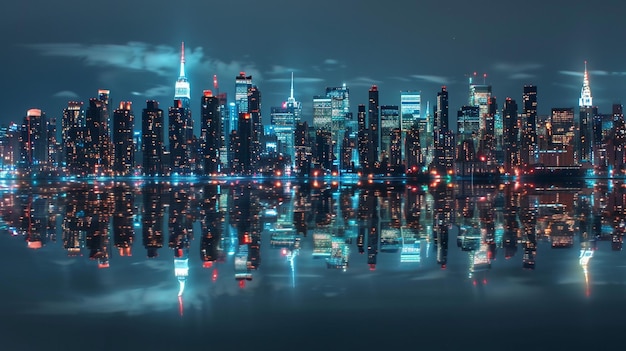The image showcases a computer-generated nighttime skyline of a large metropolitan city situated on a waterfront. Intricate high-rise buildings dominate the scene, illuminated with a variety of lights, including notable pinkish and brighter top lights that give the skyline an almost ethereal glow. A roadway runs in front of these buildings, where vivid red brake lights from traffic add vibrant reflections. The sky, obscured by teal and light blue clouds, suggests an overcast night without visible stars. The reflection of the skyline and roadway in the water below enhances the image’s colorful and dynamic atmosphere, distorted slightly to emphasize the water’s surface. Notably, a building resembling the Empire State Building stands prominently on the right, adding a recognizable landmark to the detailed, atmospheric cityscape.